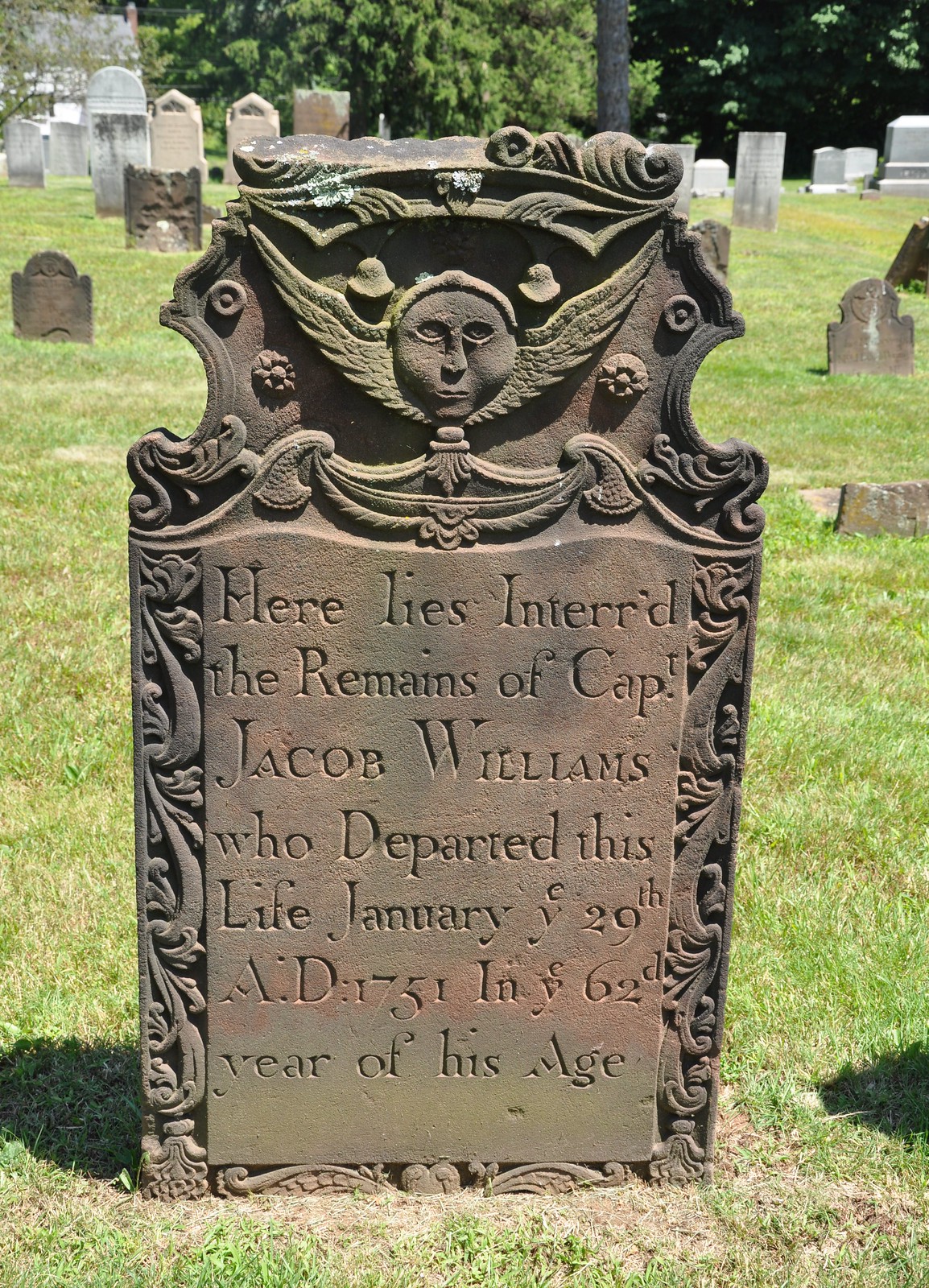In a well-kept cemetery filled with various aged and moss-covered tombstones, one prominent gravestone stands out in the foreground. The tombstone, slightly weathered but largely intact, bears the inscription: "Here lies interred the remains of Captain Jacob Williams, who departed this life January 29th, A.D. 1751, in his 62nd year of life." The tombstone features a carved face with wings at the top, adding a somber yet delicate detail. Green grass surrounds the grave, and the shadows cast by nearby trees and occasional poles enhance the serene atmosphere. Though some other tombstones in the vicinity show signs of damage, Captain Jacob Williams' memorial remains a well-preserved testament to the past.